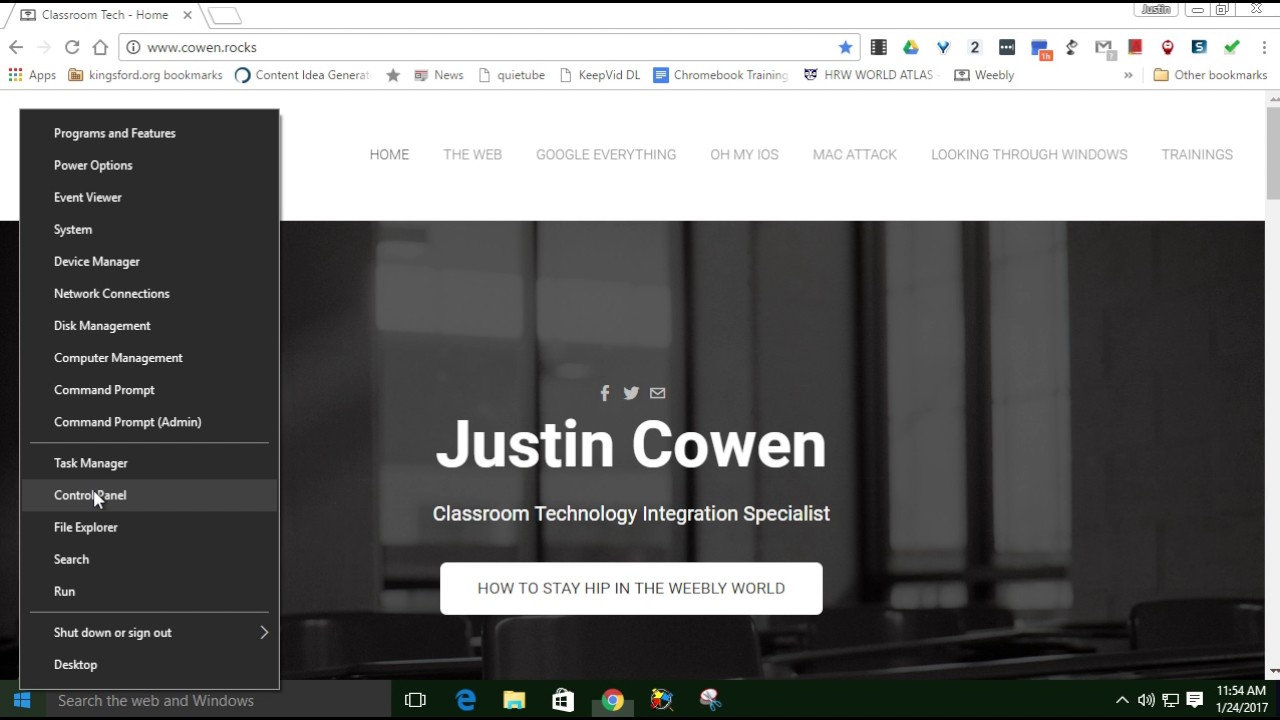This detailed screenshot captures the homepage of "Cohen.rocks," a personal website dedicated to classroom technology integration. The website belongs to Justin Cohen, who is identified as a Classroom Technology Integration Specialist. The homepage is well-organized with several clickable sections including "Home," "Web," "Google Everything," "Oh My iOS," "Mac Attack," "Looking through Windows," and "Trainings." The design showcases a professional office space image and emphasizes Justin Cohen's expertise in integrating technology within classroom settings.

A prominent text box at the bottom of the page reads, "How to stay hip in the Weebly world," suggesting guidance or tips for users. Social media icons for Facebook, Twitter, and a generic email link are available for easy contact. The taskbar at the bottom of the screen reveals it's 11:54 AM on January 24, 2017, with an indication that the user has right-clicked or left-clicked the Windows Start button and is about to click on the Control Panel.

Additionally, the screenshot reveals several bookmarks listed on the browser, including "Weebly," "HRW World Atlas," "Chromebook Training," "KeepvidDL," "QuietTube," "News," "Content Idea Generation," and "kingsford.org," suggesting the user frequently visits these sites for various educational and instructional resources.